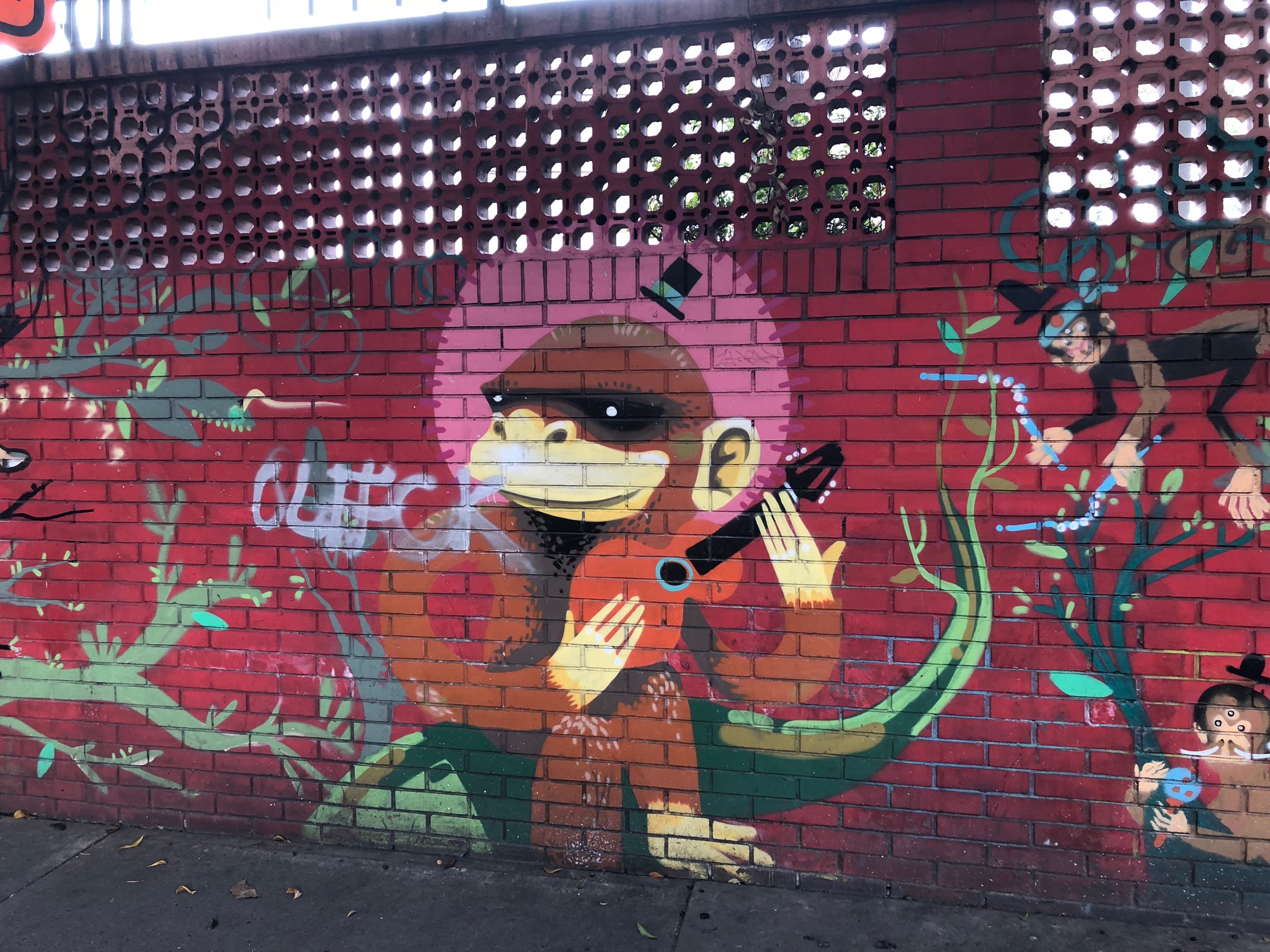This photograph features a vibrant street art mural on a red brick wall. The top quarter of the wall is composed of glass blocks with holes that allow light to pass through, while the remaining three quarters consist of solid red brick adorned with intricate graffiti. Dominating the center of the mural is a large brown monkey or chimpanzee, sitting on a branch and playing a guitar. This central figure is wearing a black and blue hat and is depicted with remarkable detail. To the right, there are two smaller monkeys situated in a tree, one of which has a notable blue headband and is holding a blue straw-like item. On the left side, various green and gray plants extend towards the central monkey, adding to the complexity of the mural. Below the brick wall, a sidewalk with scattered leaves further grounds the urban scene. There is also an enigmatic word or sequence of letters, possibly "C-L-I-F-C," to the left of the guitar-playing monkey, adding an element of mystery to the artwork.